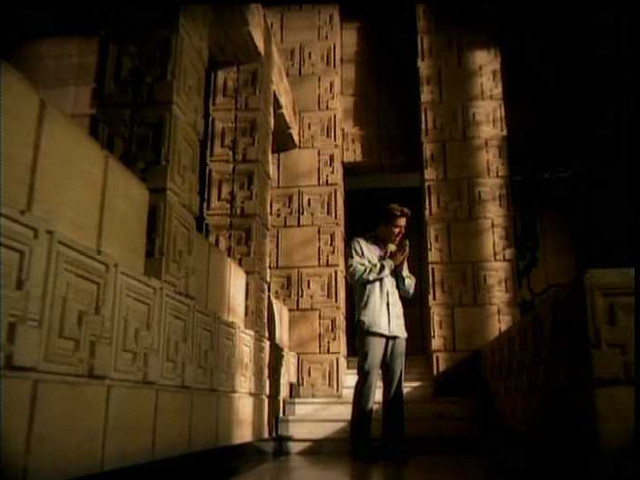A man stands in what appears to be an ancient temple, possibly reminiscent of a monastery with high, intricately carved stone walls, likely made of tan-colored limestone or sandstone. The walls, adorned with carvings, stretch high above him, framing him in the center of this vast, historical chamber. He has brown hair and is dressed in a button-down white shirt and pants, either blue jeans or gray, standing in front of a white staircase. Sunlight streams down from above, illuminating the walls, the staircase, and the man from his knees up, casting long shadows across the scene. The overall setting, with beams of natural light piercing through the darkness, gives the impression he could be praying or singing, possibly part of a music video or a scene from a movie, surrounded by an air of timeless reverence.